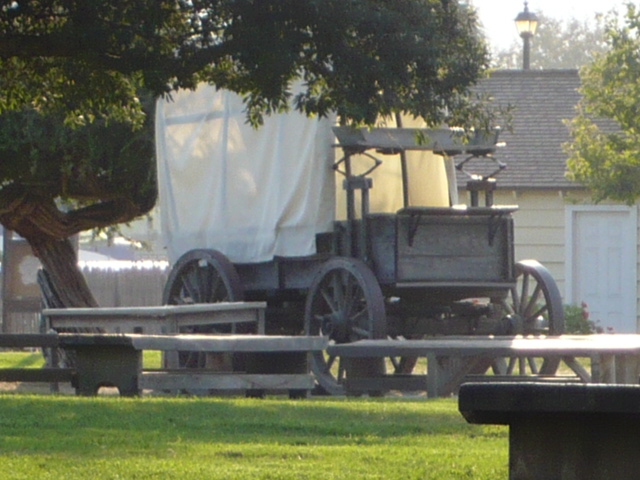In this detailed image of an Amish wagon, the scene is set in what appears to be a park with a green lawn in the forefront. The wagon, predominantly grayish-brown in color, features large wheels with prominent spokes and a white cloth cover on the back section. The wooden structure, which might be a fence or tables, stands light brownish in color and is situated nearby. Behind the wagon, a beautiful tree with a sturdy brown trunk and expansive, dark green branches stretches overhead. The background reveals a building with creamish-white siding and a slate-colored roof, contributing to the serene, park-like atmosphere. Additionally, the scene includes another tree to the right and scattered shadows, indicating the natural light filtering through the foliage and the cloth cover of the wagon. The setting, dotted with bright green grass and leafy trees, suggests it might be summertime. A small wooden fence encircles the area, and the overall image combines elements of nature with historical transportation, captured in a tranquil daylight setting.